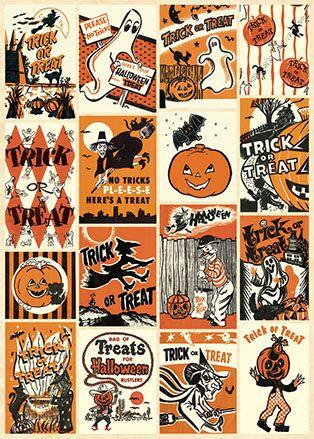The image is a vertical rectangle resembling a vintage Halloween poster, featuring a hand-drawn or hand-painted style on a yellowish beige paper. It contains a nostalgic 4x4 grid of 16 small, cartoonish Halloween-themed scenes, separated by beige lines. The color scheme is predominantly orange, black, and white, with black ink outlines. Each panel presents a unique Halloween motif including a smiling orange pumpkin, a ghost beside a "Halloween Treat" sign, a witch flying through the sky, jack-o'-lanterns, black cats, and a dancing pumpkin-headed figure with a human body. Many panels include the phrase "trick-or-treat," enhancing the festive and light-hearted mood of the artwork. The overall feel is reminiscent of collectible stamps or stickers, exuding an American nostalgic charm.